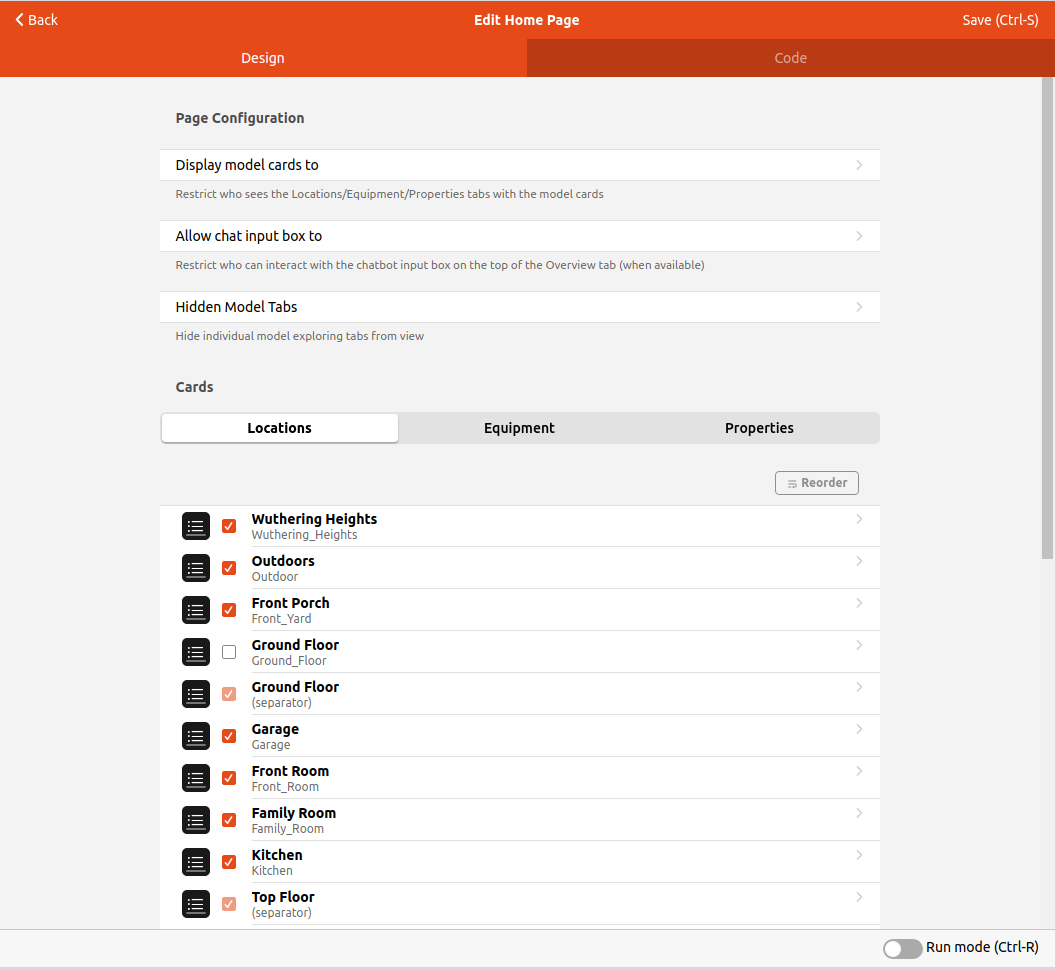This screenshot depicts a web page titled "Edit Home Page," likely for a coding or website management application. The main interface features an orange tab at the top that reads "Edit Home Page." On the left-hand side, there's a "Back" button, while on the right-hand side, there's a "Save" button, denoted with a keyboard shortcut "Ctrl + S." Below these buttons, there are two selectable tabs: "Design" and "Code," with the "Code" tab appearing to be highlighted.

The main page's background is white, with various settings and options. At the top, under "Page Configuration," there's a dropdown menu labeled "Display Model Cards To," followed by text instructing to "restrict who sees the location, equipment, and properties tabs with the model cards."

The second dropdown menu reads "Allow Chat Input Box To," with accompanying text explaining that it restricts who can interact with the chatbot input box on the top of the overview tab (when available).

A third dropdown menu, "Hidden Model Tabs," allows users to hide individual model exploring tabs from view. Additionally, the main page features a section titled "Cards," offering three options: Locations, Equipment, and Properties. The "Locations" option is highlighted with a white background, while "Equipment" and "Properties" have a gray background.

Beneath this section, there is a list of selectable items: "Weathering Heights," "Outdoor," "Front Porch," "Ground Floor," "Garage," "Front Room," "Family Room," "Kitchen," and "Top Floor." Of these, seven items are selected and marked with orange checkmarks. The "Ground Floor" item is not selected, while the "Ground Floor" and "Top Floor" selections appear with a slightly dimmed checkmark color.

Overall, the page provides detailed and configurable options for managing what elements are displayed and who can interact with various components of the home page.